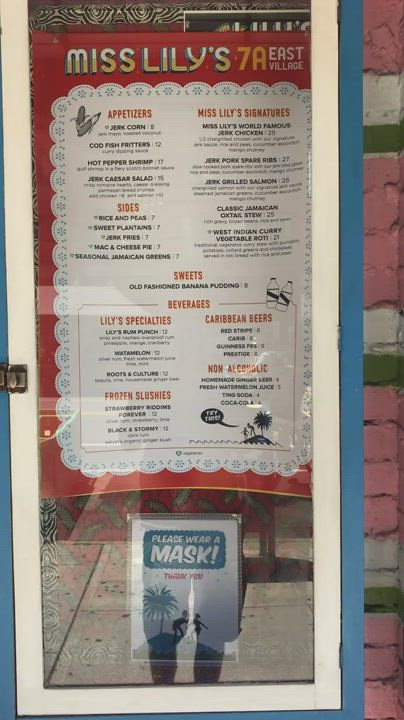The image features a white door with a glass panel in its center, flanked by light blue walls. Adjacent to the door, a brick wall showcases a mix of colors: the top section is red, followed by alternating stripes of white and green. This colorful pattern continues with segments of red, white, green, and reddish hues.

The top part of the glass door features a zebra print design. Above the door, there is a red rectangular sign that reads "Miss Lily's 7A East Village." On top of this sign, a large white doily-like rectangle is displayed. In the middle of the doily appears to be a menu with "Appetizers" written in red, followed by black text that is not fully legible. Further down, there are sections labeled "Sides," "Miss Lily's Signatures," "Sweets," with corresponding item descriptions in black text. The menu also has a section for "Beverages," outlined in red with two bottle illustrations on the upper right corner.

Additionally, the menu lists "Lily's Specials," "Frozen Slushies," "Caribbean Beers," and "Non-Alcoholic" options, each highlighted in red with further details in black text. On the lower half of the image, an illustration of an island with a tree and two people is surrounded by a black speech bubble containing small white text, with wave designs encircling the island.

Below this, a poster with a clear plastic border and a white center is displayed. It contains a large blue rectangle featuring the words "Please Wear a Mask" in white, followed by "Thank You" in red, and includes a depiction of the same island scene with two people and a tree.